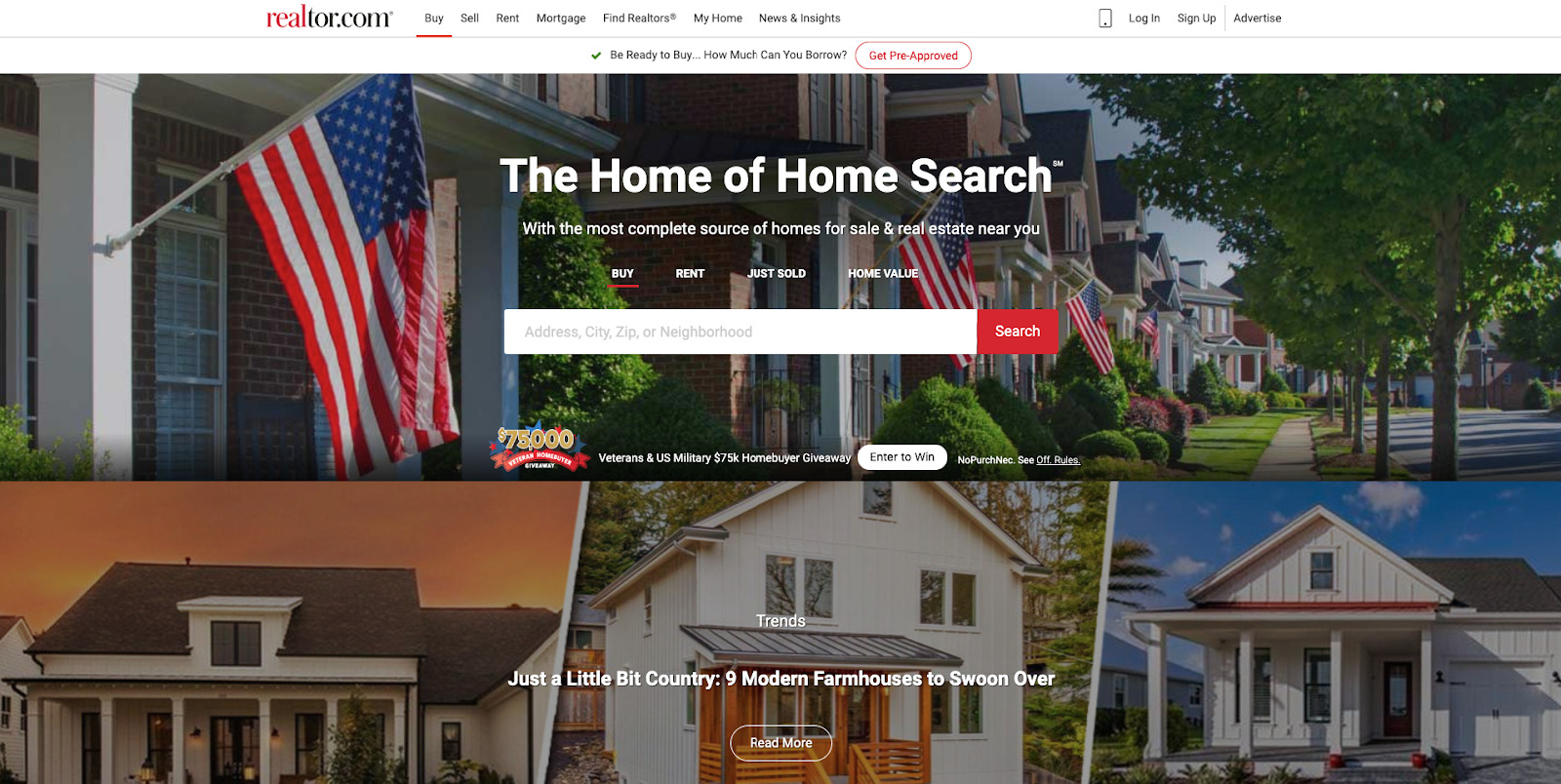The image is a web page for buying real estate on Realtor.com. On the upper left side, not fully in the corner but towards the left, there is red and black text that reads "Realtor.com." In the center of the image, white text proclaims, "The Home of Home Search," and below that, in smaller white text, it says, "With the most complete source of homes for sale and real estate near you." Beneath this statement are four categories: Buy, Rent, Just Sold, and Home Value, with the Buy category selected, indicated by a red underline.

A search bar is positioned under these categories, containing gray placeholder text that suggests search criteria such as "Address, City, Zip, or Neighborhood." The website features images of houses throughout the background. The top half of the image displays a residential neighborhood with houses closely spaced together, while the bottom half showcases three distinct houses set in different environments, highlighting the website's diverse range of real estate listings.